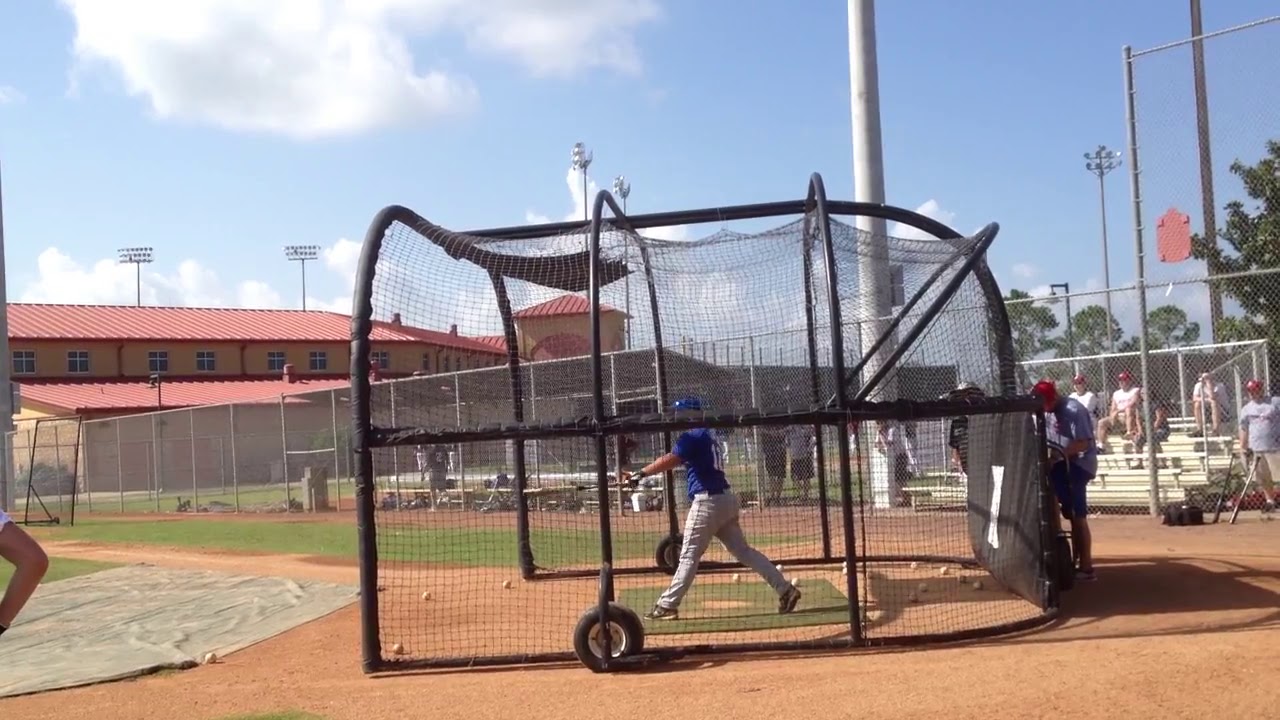In this vibrant, outdoor scene captured during the day, a baseball player in a blue jersey, blue helmet, and gray pants is taking batting practice inside a mesh batting cage designed to keep stray balls from hitting spectators. Positioned in the foreground on the brown soil of the infield, the player is stretching with his bat extended in his left hand, preparing for a pitch. Green grass surrounds the infield area, and a gray tarp is visible on the ground in front of the cage.

Behind the player, a tall chain-link fence guards a set of bleachers, where a few spectators, some in red caps, are seated. The image also captures part of another person's arm in the bottom left corner. In the background, a large red-roofed, beige building with a gable is visible, accompanied by a distinctive gabled tower and several light poles. The scene is bright and sunny, with a blue sky scattered with white, fluffy clouds overhead, adding a serene backdrop to the bustling baseball environment.